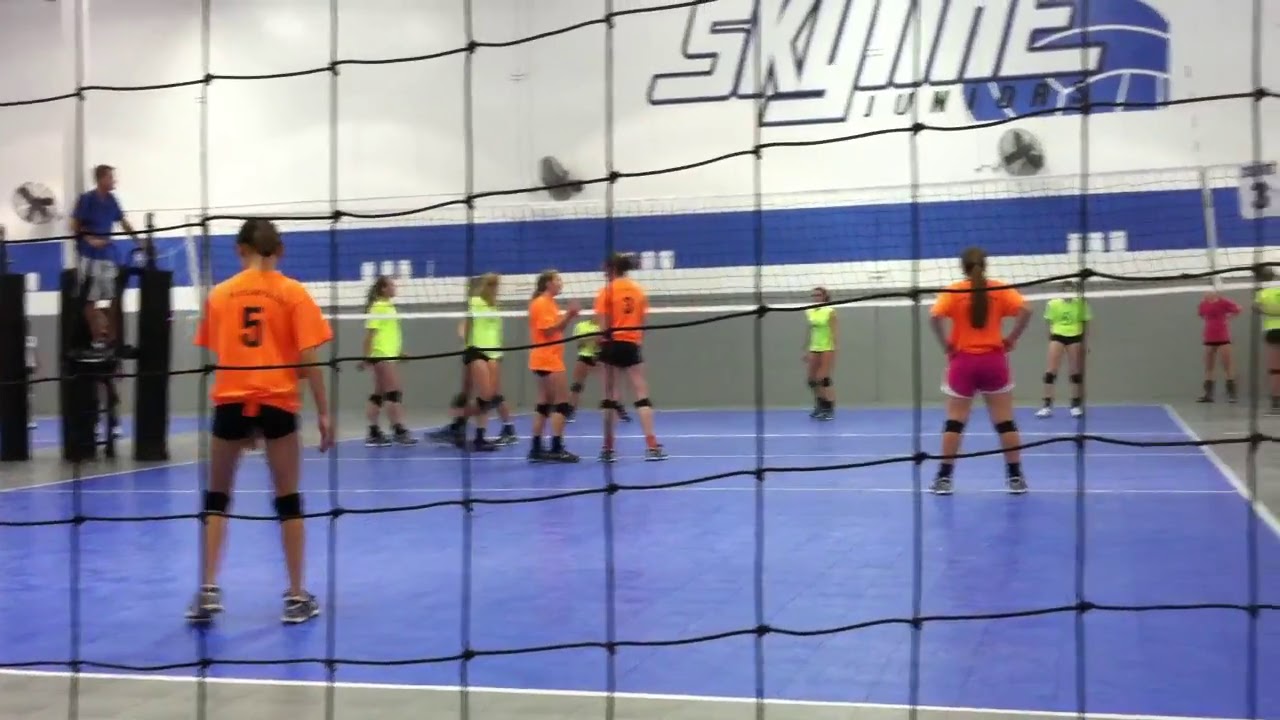The photograph captures an intense volleyball game viewed from behind a black net, which slightly obscures the scene. The blue court is painted with white lines and surrounded by a gray perimeter. Dominating the foreground is a team in bright orange shirts with black knee pads and shorts. One player, with the number 5 on her shirt, is centrally located, her back turned to the camera, wearing gray shoes and contrasting her teammates, one of whom is sporting purple shorts instead of black. Towards the left, another player in an orange shirt, number 3, stands near the net. In the background, their opponents wear fluorescent green shirts with black shorts and knee pads, preparing for their next move. A referee, dressed in a blue shirt and gray shorts, is elevated on a platform on the far left, overseeing the match. The back wall features a mural with the words "Skyline Juniors" and a painting of a blue volleyball, framed by three large fans that help circulate the air in the gym. The combination of distinct team uniforms, the court’s vivid colors, and the detailed backdrop offers a dynamic and immersive view of the volleyball match in progress.